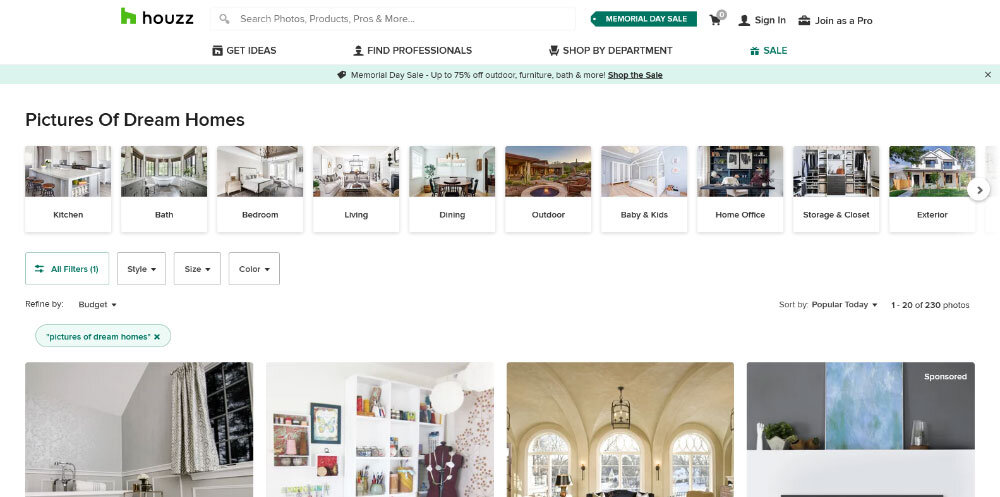Certainly! Here's a detailed description based on the provided information:

---

The image portrays the homepage of a website dedicated to house-related resources, prominently featuring the logo in the upper left corner with a green house icon next to the name "Houzz" spelled as H-O-U-Z-Z. Adjacent to the logo, there is a versatile search bar offering options to look up photos, products, professionals, and more. A noticeable green banner announces a "Memorial Day Sale," followed by icons for a shopping cart and options to sign in or join as a professional.

Beneath the initial banner, there are four main navigation options: "Gift Ideas," "Find Professionals," "Shop by Departments," and "Sale." A secondary, light green banner emphasizes the "Memorial Day Sale," advertising up to 75% off on outdoor furniture, baths, and more, with the text "Shop the Sale" highlighted in bold and underlined, suggesting a clickable link.

The section below features a white background with the header "Pictures of Dream Homes" in black text. This area is organized into a horizontal column showcasing various categories of interior and exterior home images. Categories include Kitchen & Bath, Bedroom, Living, Dining, Outdoor, Baby & Kids, Home Office, Storage & Closet, and Exterior. A rightward arrow indicates the availability of more categories to explore. Each category provides a selection of dream home visuals for specific areas, enhancing user convenience.

Additionally, filter options are available, allowing users to refine their search based on style, size, or color. The bottom portion of the page appears to present an extended array of home images, further enriching the browsing experience.

---

I hope this meets your needs! If you have any specific elements you'd like to emphasize or any additional details to add, please let me know.